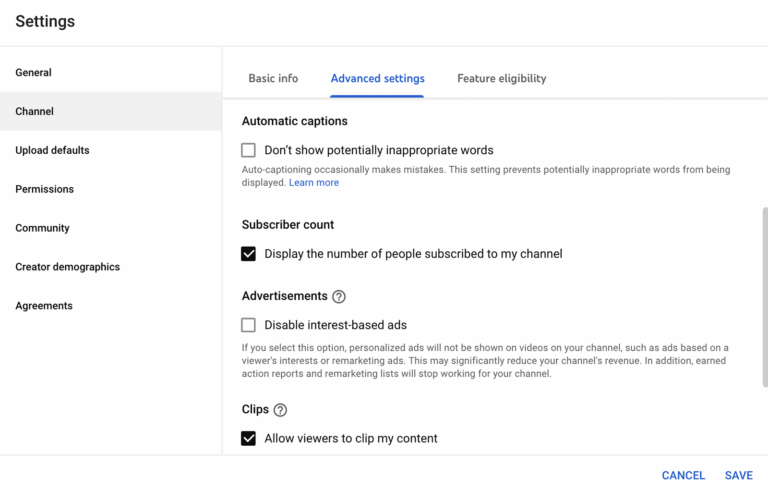This is a detailed screenshot of an open settings menu from a content management platform. The background of the menu is white, with the word "Settings" prominently displayed in the top left corner. Below "Settings," there is a vertical list of clickable options which include: General, Channel, Upload Defaults, Permissions, Community, Creator Demographics, and Agreements. The "Channel" option is currently selected, highlighted with a gray rectangle, indicating that this section is active.

On the right side of the screen, the channel settings are displayed, divided into three subsections: Basic Info, Advanced Settings, and Feature Eligibility, all labeled in gray font. The user has selected "Advanced Settings," which is now highlighted in blue and underlined, showing it is the active subsection.

Within the "Advanced Settings" menu, the first option listed is "Automatic Captions." Accompanying this option is a check box, labeled "Don't show potentially inappropriate words." There is a brief explanation beneath this: "Auto captioning occasionally makes mistakes. This setting prevents potentially inappropriate words from being displayed." Next to this explanation, there is a clickable "Learn More" link, highlighted in blue.

Below the "Automatic Captions" section, the menu provides the option to display the channel's "Subscriber Count." The check box for this option is selected, showing a black box with a white check mark. The descriptive text beside it reads: "Display the number of people subscribed to my channel."